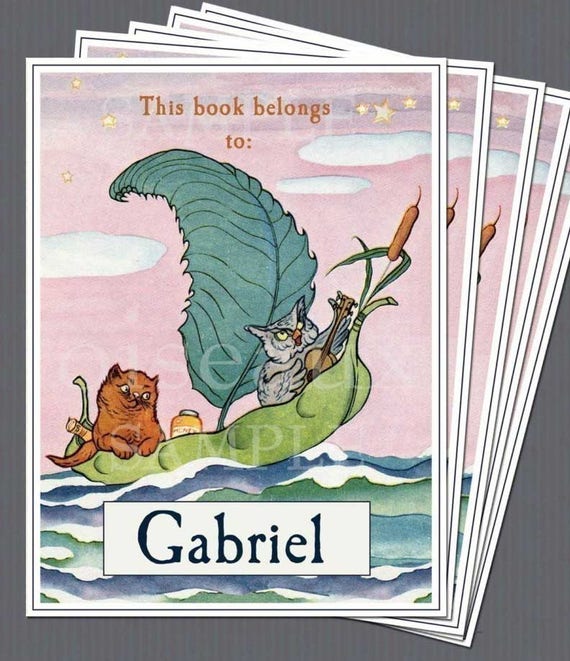On a grey surface, there are several overlapping card-like sheets, with the topmost card featuring a detailed, whimsical illustration. At the center of the card, animals are depicted sailing in a boat crafted from a large green leaf. The boat carries a brown cat on the left and a grey owl on the right, the latter playing a stringed instrument, possibly a banjo or a guitar, with its wings. In front of the cat is a yellow jar, and a large leaf serves as the sail. A cattail plant adorns the top of the boat image. The sky above is a pink hue, dotted with yellow stars and greyish-white clouds. At the top of the card, text reads, "This book belongs to..." and at the bottom, the name "Gabriel" is printed in bold black letters against a white background. The illustration also features translucent grey watermarks that are barely legible.